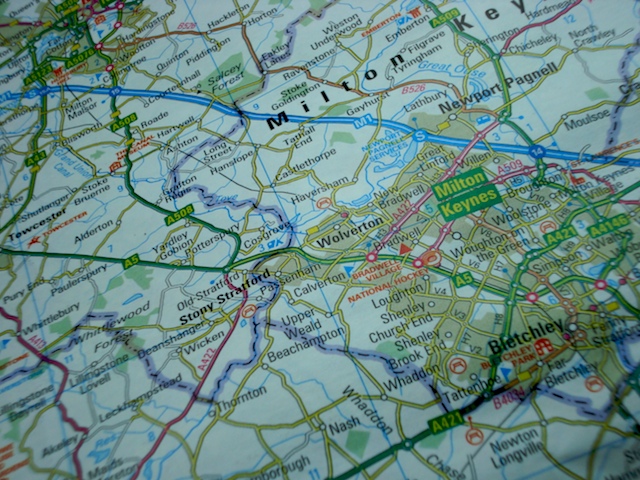This detailed image shows a close-up photograph of a road map with a light tan, beige background. The map prominently features the large area of Milton Keynes, along with several surrounding towns including Bletchley, Newport Pagnell, Wolverton, Old Stratford, and Stony Stratford. Numerous lines in various colors—green, red, purple, yellow, and blue—crisscross the map, representing different roads and transportation routes. Notably, a blue-marked road, possibly labeled M1, runs through the map. The text on the map is small and varies in color, with names of places such as Milton Keynes and Bletchley appearing in formats like black text, red text, and yellow-on-green boxes. The map also shows open green areas suggesting fields and darker gold shades indicating denser urban regions. The angled shot of the map, not typical of online maps, gives it a more tactile, possibly printed appearance.